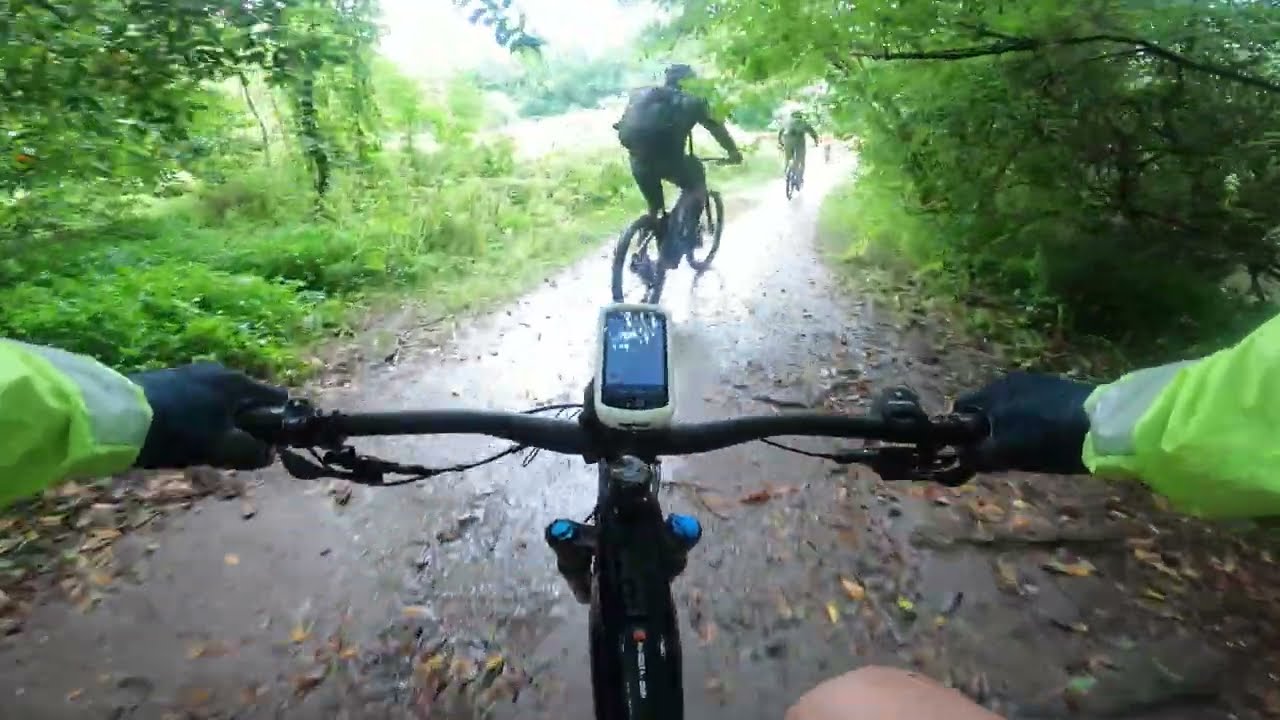This outdoor daytime image captures a first-person view of a bicycle rider on a wet, dark gray or brown paved trail, enveloped by an abundance of trees and overgrown shrubbery. The rider is wearing black gloves and a long-sleeve top (green or yellow) paired with shorts, revealing a bare right knee. Their black bike features a phone or GPS device mounted at the center of the handlebars, which also display the grips, brake levers, and front forks. The perspective reveals two other cyclists ahead on the slightly shadowed trail, dotted with dead leaves and puddles, suggesting it just rained. Sunlight gleams down from the left, casting a bright but blurred illumination onto the scene.